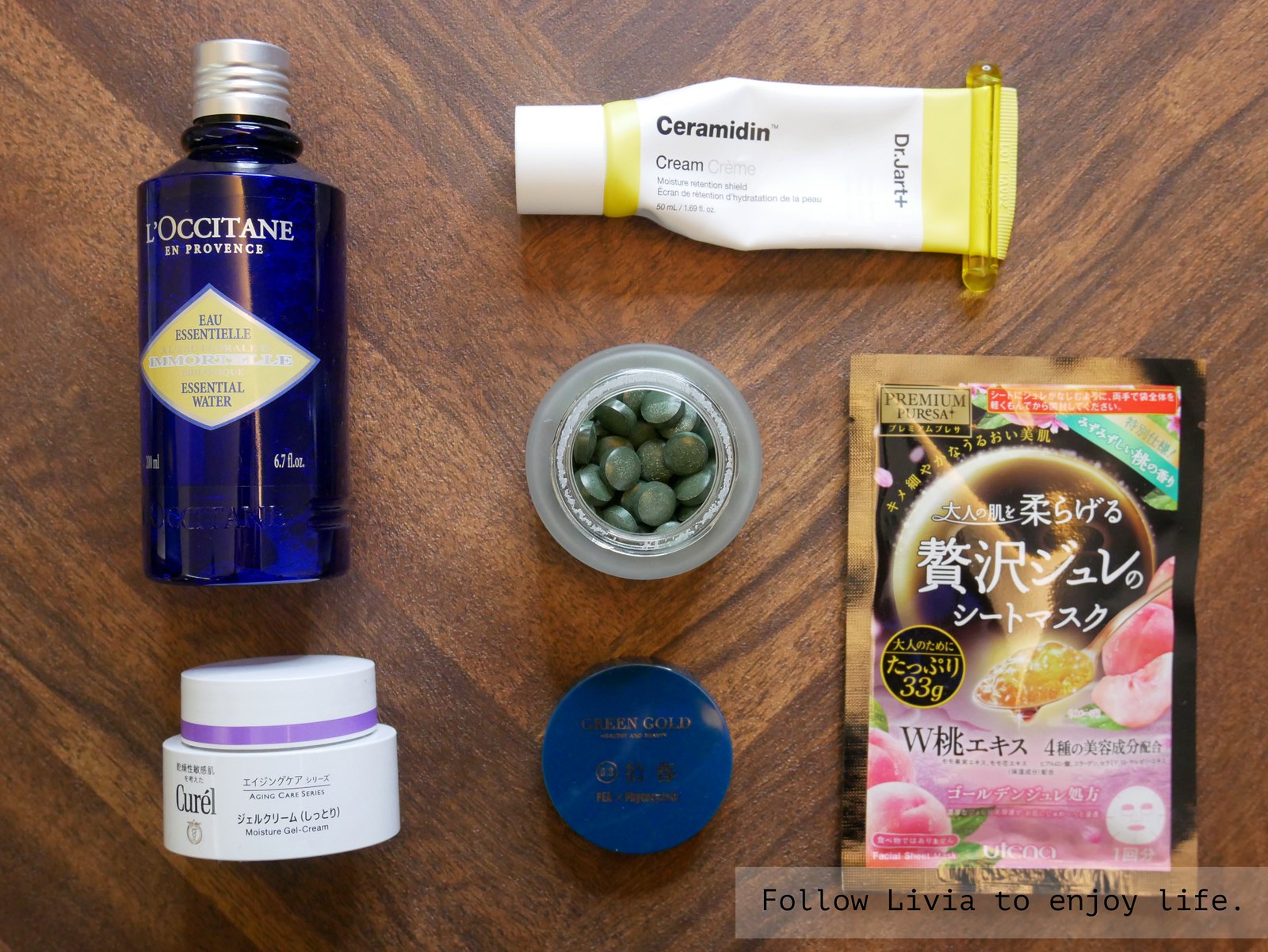This photograph showcases an array of skincare products arranged on a wood-grain tabletop with a chevron pattern of light and dark brown tones. 

In the bottom right-hand corner, a gray box bears the text "follow Livia to enjoy life" in black. Among the skincare items, positioned in the upper left is a blue bottle with a silver cap labeled "Le Osteen en Provence, A Essentiel Essential Water, 6.7 fluid ounces." 

To the bottom left, there is a short cylindrical white container with a purple-bordered lid. This is marked as "Curel Aging Care Series Moisture Gel Cream."

At the top, a white tube resembling a toothpaste container features a yellow plastic piece at the end for squeezing out the product. This tube, bordered by yellow with a white cap, is labeled "Ceramidin Cream, Dr. Jart Plus."

Next, there is a clear container filled with green tablet-like pills, topped with a blue lid that reads "green gold."

To the far right, there is a face mask package in gold and black, featuring Japanese lettering. The packaging is adorned with pink fruit illustrations and shows a white face image with cutouts for the eyes and mouth.

The detailed textures and colors of the products and the tabletop create a visually engaging and organized display.